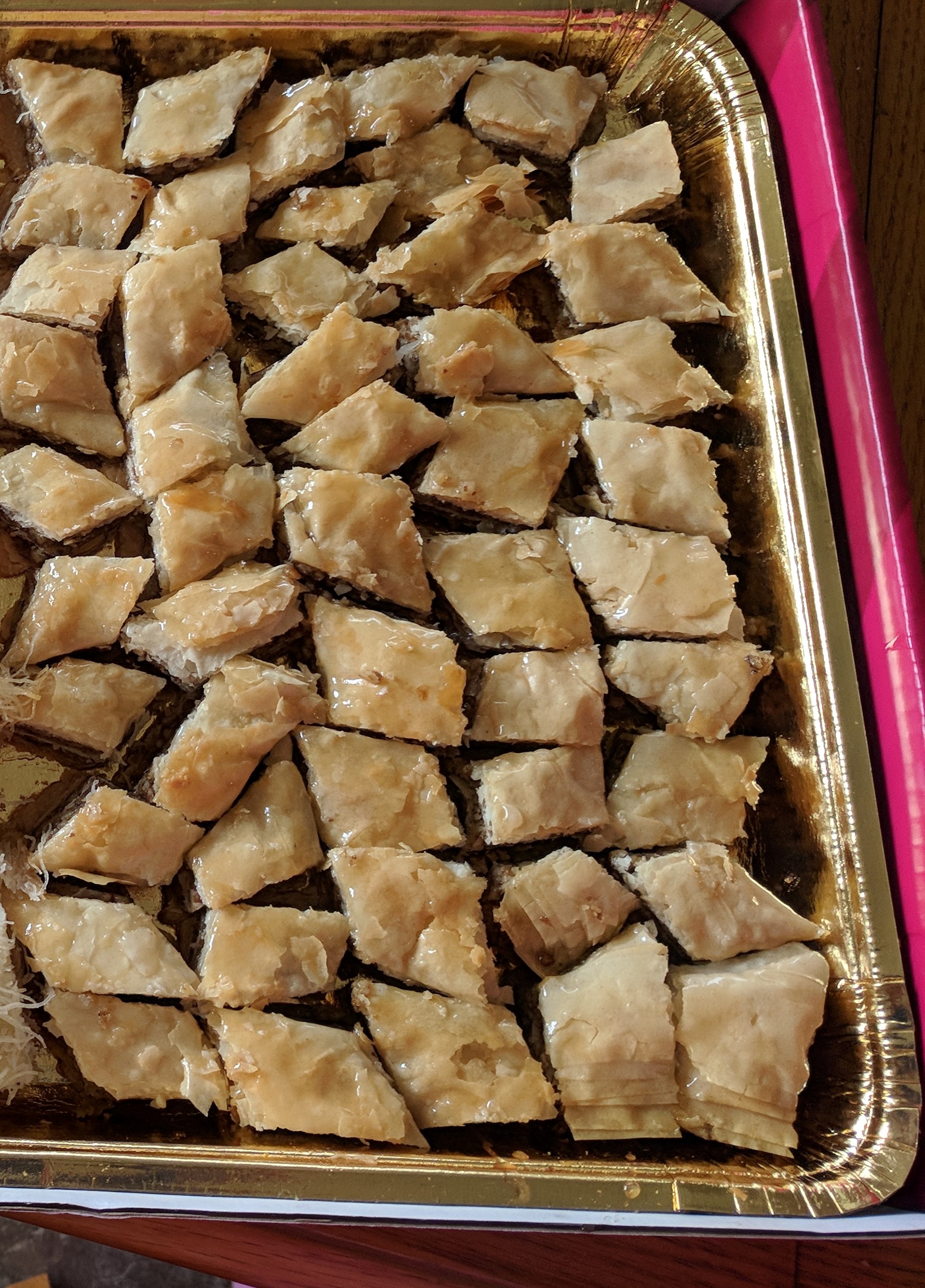The image depicts an overhead shot of a silver aluminum foil pan filled with a dessert that appears to be baklava. The pan, which is approximately 13 by 9 inches in size, sits inside a pink cardboard box, visible on the right side of the image. The dessert is cut into diamond-shaped and rectangular pieces, arranged neatly rather than piled atop one another. The baklava pieces are light tan to almost white in color, with a distinct gleam on their surface suggesting a syrup glaze. The foil pan has a thin blue outline on the bottom, and the scene is set on a dark, cherry-colored wooden table, with portions of the table visible at the bottom and the upper right corner of the picture. The background overall is dark, with some gray shading at the bottom left. There is no text in the image, and the setting gives the impression of being in a restaurant or bakery.